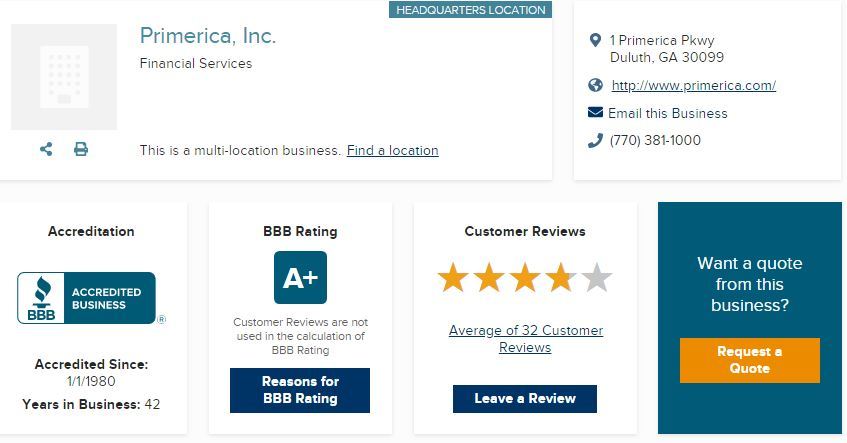In the image, a detailed layout of the company's information is presented in a structured and organized manner, highlighting various aspects of its business profile and ratings.

**Top Section:**
- **Top Left:** The label reads "Primerica, Inc., Financial Services."
- Immediately to its left is a gray square featuring a white square in its center adorned with gray dots. 
- Below this grey square are a share icon and a print icon.
- **Top Center:** The text states, "This is a multi-location business," with an underline emphasizing the word "Location."
- **Top Right:** Noted as "Headquarters Location" against a blue background.
- The full address is listed as "1 Primerica Parkway, Duluth, Georgia 30099."
- Below the address is a link to the company's website, followed by an email address for the business, and a phone number.

**Bottom Section:**
- **First Label (Left):** Designated for "Accreditation," it states, "Accredited Business since January 1st, 1980," and notes, "Years in Business: 42."
- **Second Label (Center Left):** Displays the "BBB Rating" as A+.
- Below the rating is a dark blue button with white text indicating "Reasons for BBB Rating," which users can click on for more information. 
- **Third Label (Center Right):** Dedicated to "Customer Reviews," showing a current rating of approximately 3.9 out of 5 stars, with the fourth star illuminated in gray.
- It mentions, "Average of 32 customer reviews," along with a prompt to "Leave a Review" followed by a dark blue button.
- **Fourth Label (Right):** Promotes getting a quote from the business, appearing in white text within a blue square, below which is an orange rectangle with the text "Request a Quote" centered within it.

This comprehensive layout provides a clear and detailed overview of Primerica, Inc.'s business credentials, location, and customer feedback.